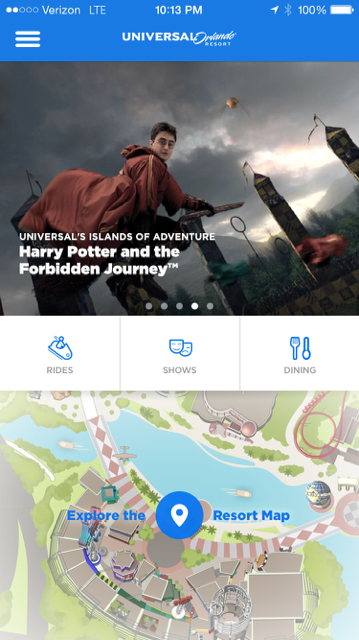This image depicts a scene on a mobile phone screen showcasing the Universal Orlando Resort app interface. At the top of the screen, set against a blue background, is the app's title, "Universal Orlando Resort." The status bar indicates the phone is connected to Verizon LTE with full signal strength, reads 10:13 AM, and has a 100% battery charge.

Dominating the main portion of the screen is an advertisement for "Harry Potter and the Forbidden Journey" attraction, located within Universal's Islands of Adventure. The image features Daniel Radcliffe as Harry Potter flying on a broomstick with a stormy, gray backdrop that likely emulates a scene from the Harry Potter movies.

Below this, there are three navigation buttons labeled "Rides," "Shows," and "Dining," each accompanied by hand-drawn style icons. The "Rides" button features a person in a ride vehicle, the "Shows" button shows the traditional comedy and tragedy masks, and the "Dining" button displays a fork and spoon.

At the bottom of the screen, there is a call-to-action section prompting users to "Explore the Resort Map," which displays a cartoonish-style map of the resort. The map highlights various attractions with emphasis on a large blue circle in the center, likely signifying a point of interest.

Additionally, at the top-left corner of the screen are three horizontal lines indicating a menu option for accessing further features and options within the app.